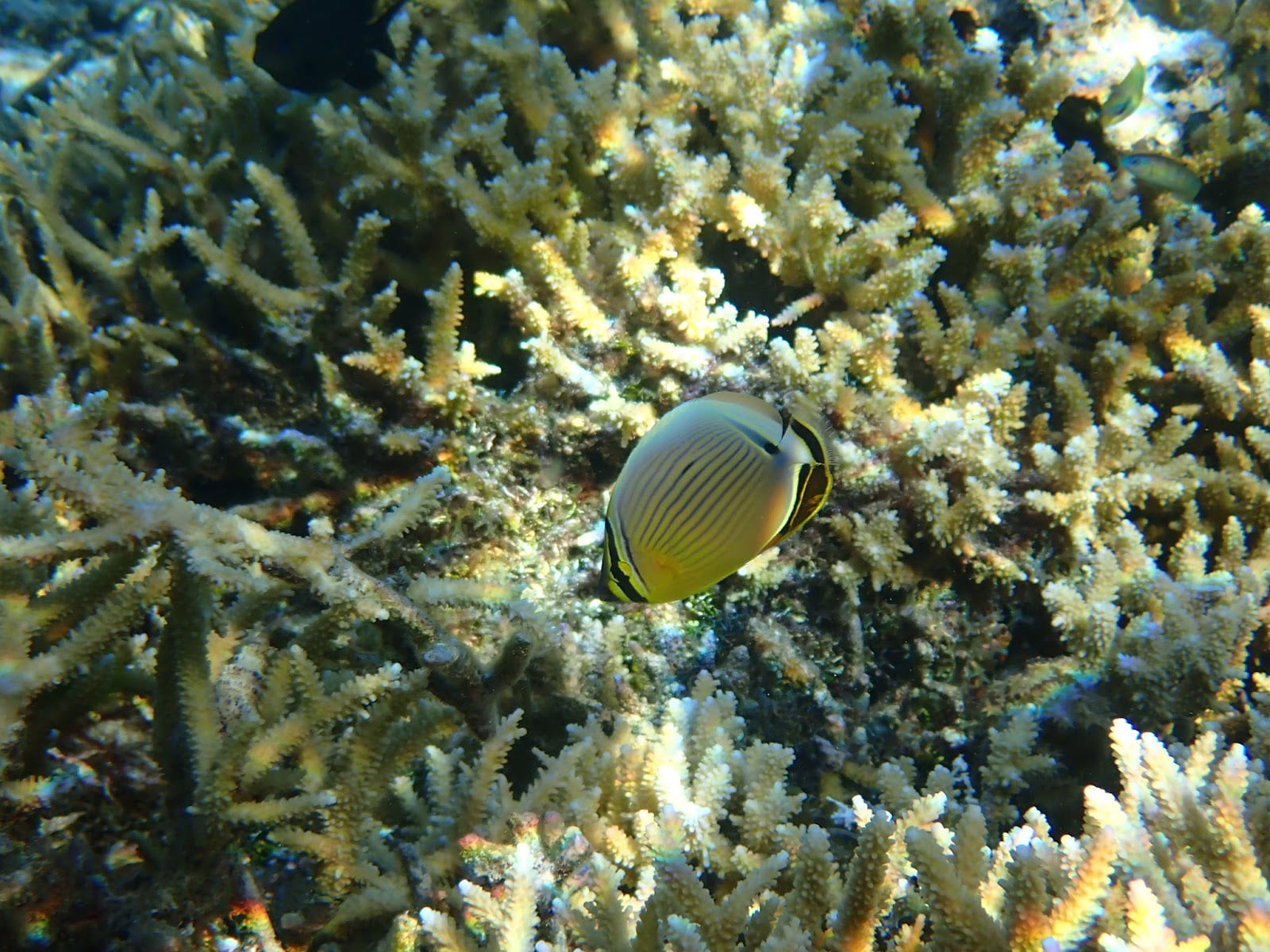This underwater photograph captures a vibrant scene amidst a coral reef. Central to the image is a striking yellow, flat fish adorned with distinctive black stripes running horizontally down its body, tapering toward its black and yellow striped tail fin. A notable black strip runs vertically across its face, accentuating its yellow eye, as it directs its gaze downward at the white corals beneath. The coral itself has a homogenous structure, resembling small fingers, with some pieces reflecting a rainbow-like glare from the sunlight above. In the top left corner, a larger, dark-hued fish resembling a black goldfish can be seen. The overall lighting and clarity suggest that the photo was taken during a scuba diving excursion in relatively shallow waters, where sunlight can penetrate and illuminate the scene vividly.